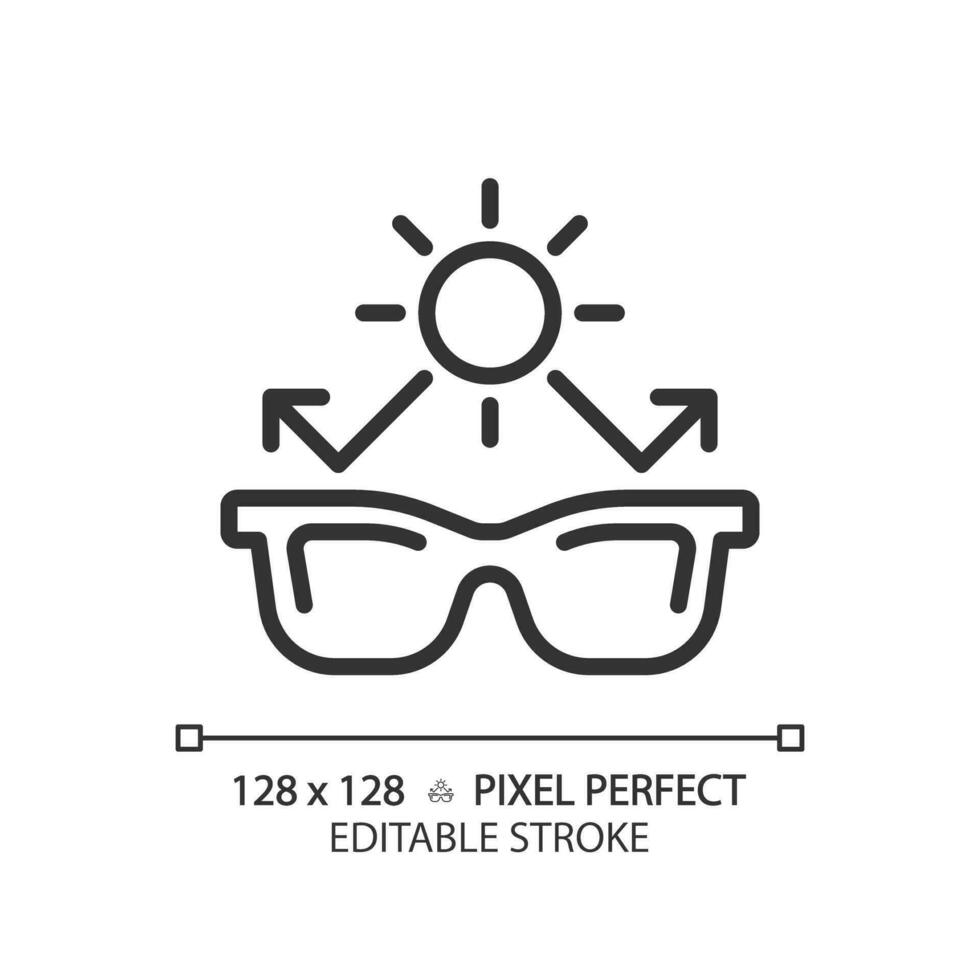This image is a minimalistic black line drawing on a white background, likely designed as an icon. At the bottom, it reads "128 by 128 pixel perfect, editable stroke," and features a thin black line running horizontally with small squares at each end. Above this line is a pair of eyeglasses with thick black rims, simplified to the extent that the lenses are only suggested by lines at the top outside corners of the frame, forming a sideways L-shape. Positioned just above the glasses is a circular design representing a sun, complete with rays depicted by short lines radiating outward. Two of these rays extend down to the glasses, where they appear to reflect off the lenses and continue outward at 90-degree angles, terminating in arrowheads. The layout and style suggest this could be clipart for sunglasses or UV protection glasses, emphasizing clarity and editability.